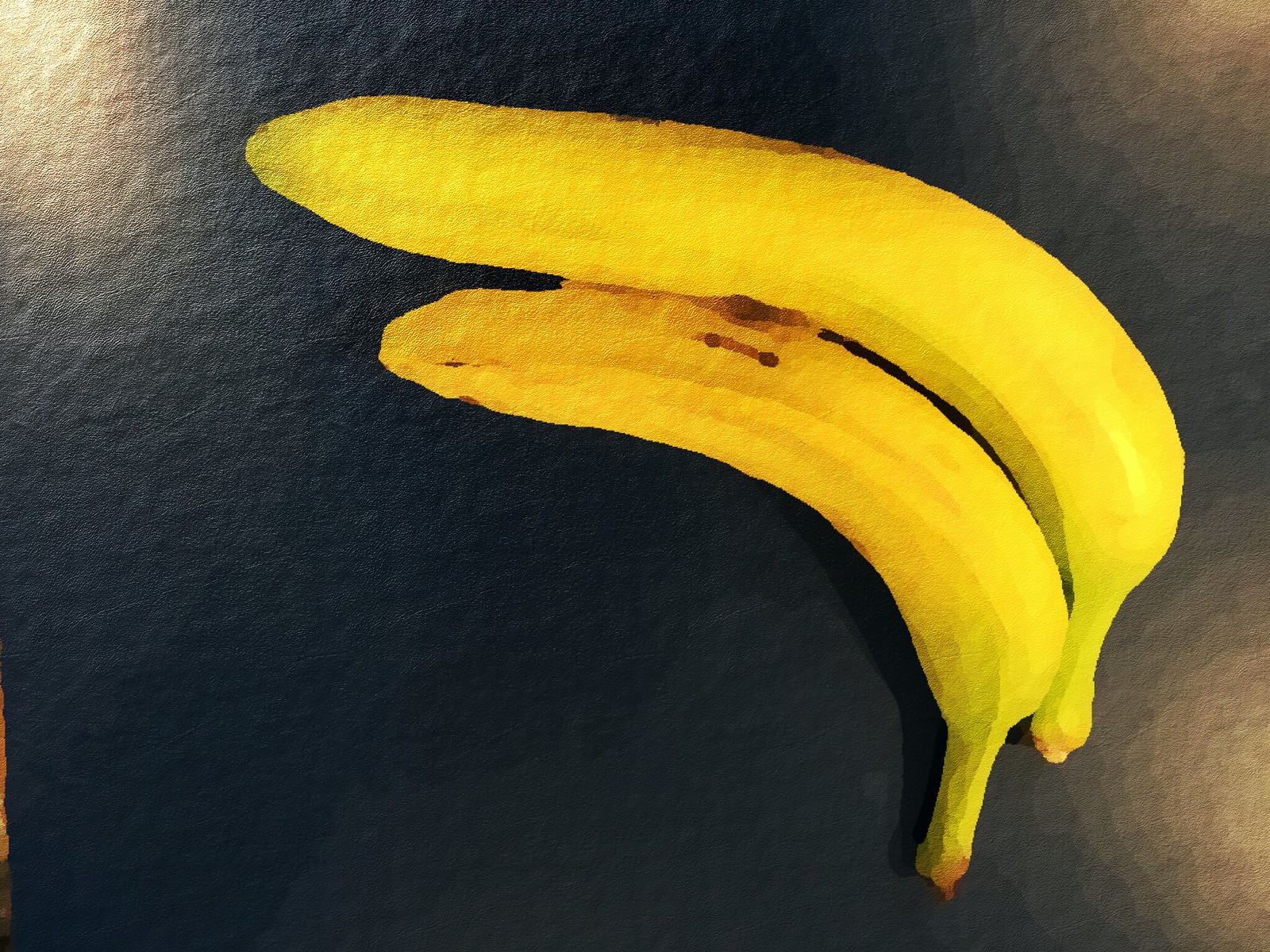This detailed caption is descriptive of the combined key elements from the three captions:

A close-up, stylistically colored painting depicts two bananas against a predominantly black background. The composition features light beams emanating from the upper left and right corners, as well as the bottom right corner, creating an artistic glow around the fruit. The painting employs yellows with brown streaks and hints of light green near the stems for shading. The two bananas, which are not attached to each other, form an inverted crescent shape, with the larger banana curving over the smaller one. The smaller banana has a small scar along its lower end. Some filters appear to have been used to enhance the painting, giving the image a non-realistic, artistic feel, as if viewed under special lighting, adding to the unique visual impact. The bananas themselves occupy about 50 to 60% of the landscape-oriented image.